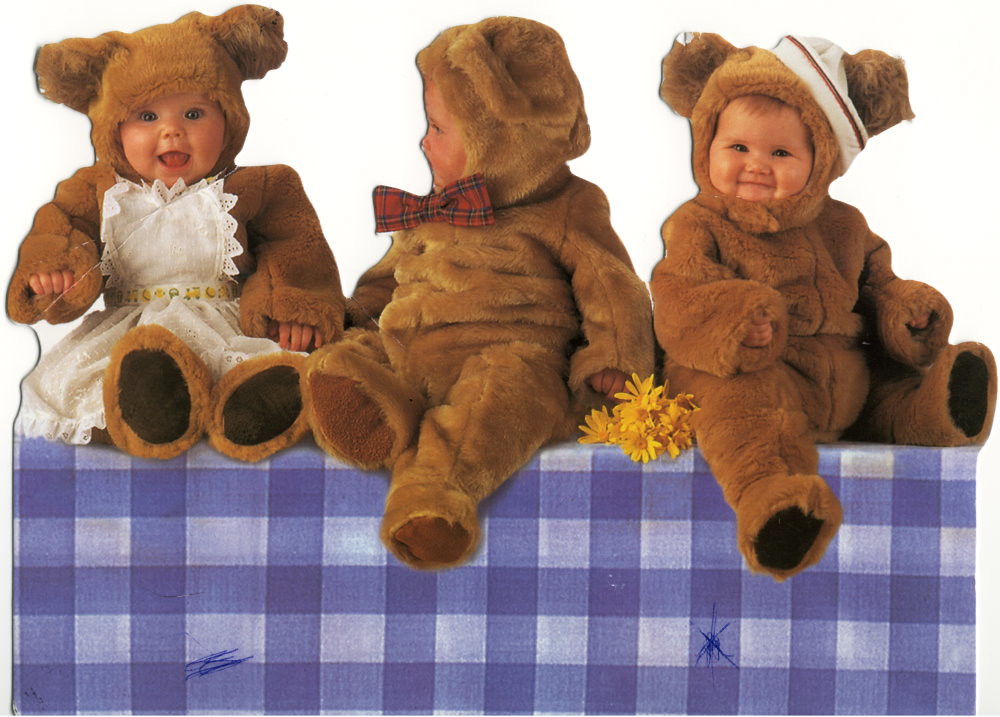This photograph showcases three adorable infants, all dressed in light brown teddy bear costumes, sitting on a blue and white checkered tablecloth, which appears to be drawn on with ink pen scribbles. The background is plain white, enhancing the focus on the children and their charming outfits. The baby on the left has a fluffy teddy bear costume with an elaborate white apron featuring a scalloped edge and a belt with yellow markings, looking straight ahead. The middle infant, also clad in a bear costume, is turned towards the left, revealing a red and green bow tie. This baby holds a bouquet of yellow daisies, positioned between them and the third child. The infant on the right, facing the camera with a big smile, sports a similar bear suit adorned with a jaunty sailor's cap, which has a slit for the left ear. The scene is reminiscent of an Ann Geddes classic, capturing the innocence and playful spirit of these little ones.